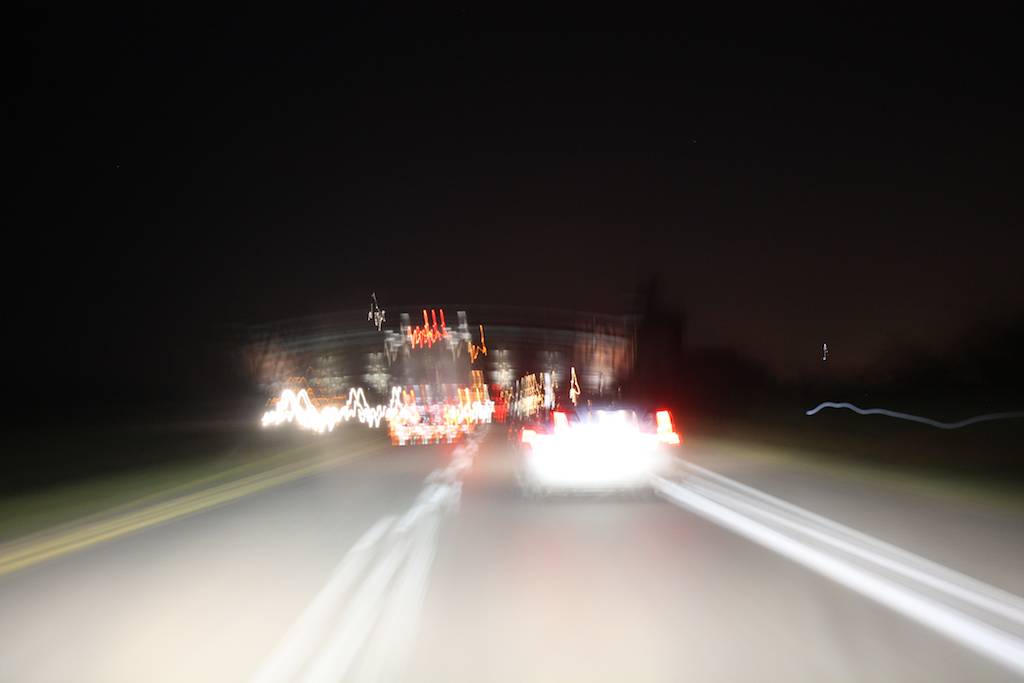A nighttime image of a highway blurred by an astigmatic effect, mimicking the perspective of a driver with poor vision. The highway appears to be an interstate, with the vehicle in the right-hand lane and an oncoming lane visible, though obscured by the blurry surroundings. To the side, a patch of grass or unpaved shoulder can be seen, adding to the indistinct scene that might suggest a potential merger situation. Ahead, a series of duplicate and unclear shapes indicate the presence of a convoy of 18-wheeler trucks, their forms rendered indistinguishable by the overlapping blurs of the headlights and taillights, contributing to the overall sense of visual disorientation.